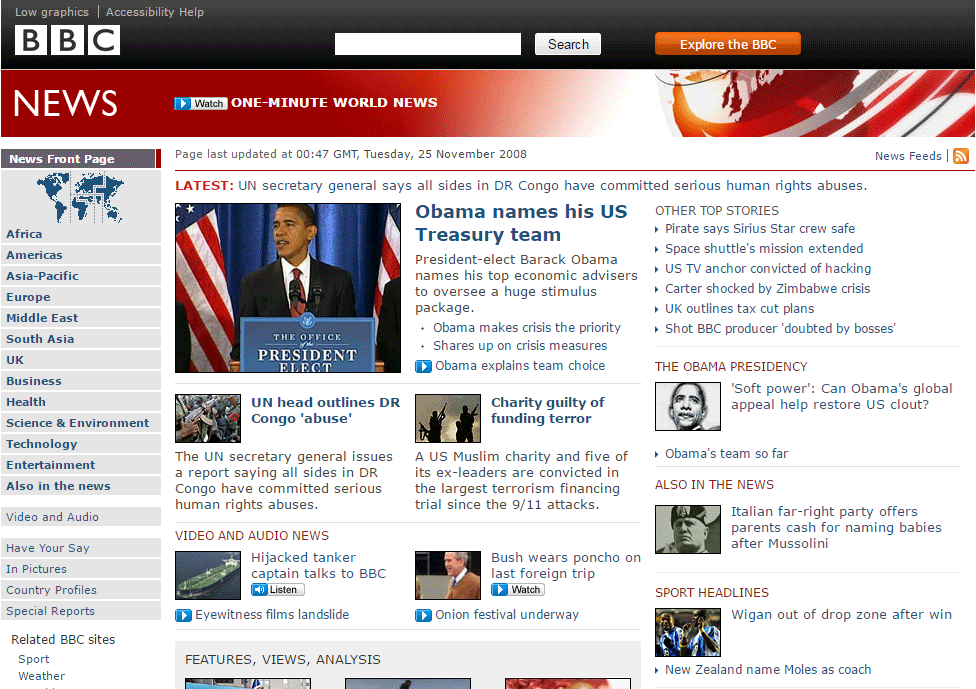The top of the image features a long black bar with the text "Low Graphics | Accessibility Help" aligned to the left. Below this bar, white blocks spell out "BBC." Adjacent to these blocks is a search bar with the word "Search" displayed in a gray box. Next to the search bar, an orange box contains the phrase "Inside, explore the BBC." Directly beneath this is a red banner with "News" written in white text. There is an option to click and watch the "One-minute World News."

The main section of the page showcases an image of Barack Obama standing at a podium with the American flag draped behind him. A blue box on the podium reads "The Office of the President-elect." To the right of this image is a headline stating, "Obama names his U.S. Treasury team." Above this headline, it mentions that the page was last updated at 00:47 GMT on Tuesday, 25th November, 2008.

Below Obama's image, another image depicts silhouettes of people holding guns, accompanied by the text "Charity guilty of funding terror." Further down, an image of President Bush wearing a brown jacket is displayed with the caption "Bush wears poncho on last foreign trip."

To the right, there are two black and white images: one of Barack Obama and another of a soldier. The bottom section of the page features sports headlines, specifically noting, "WIGAN out of drop zone after win."